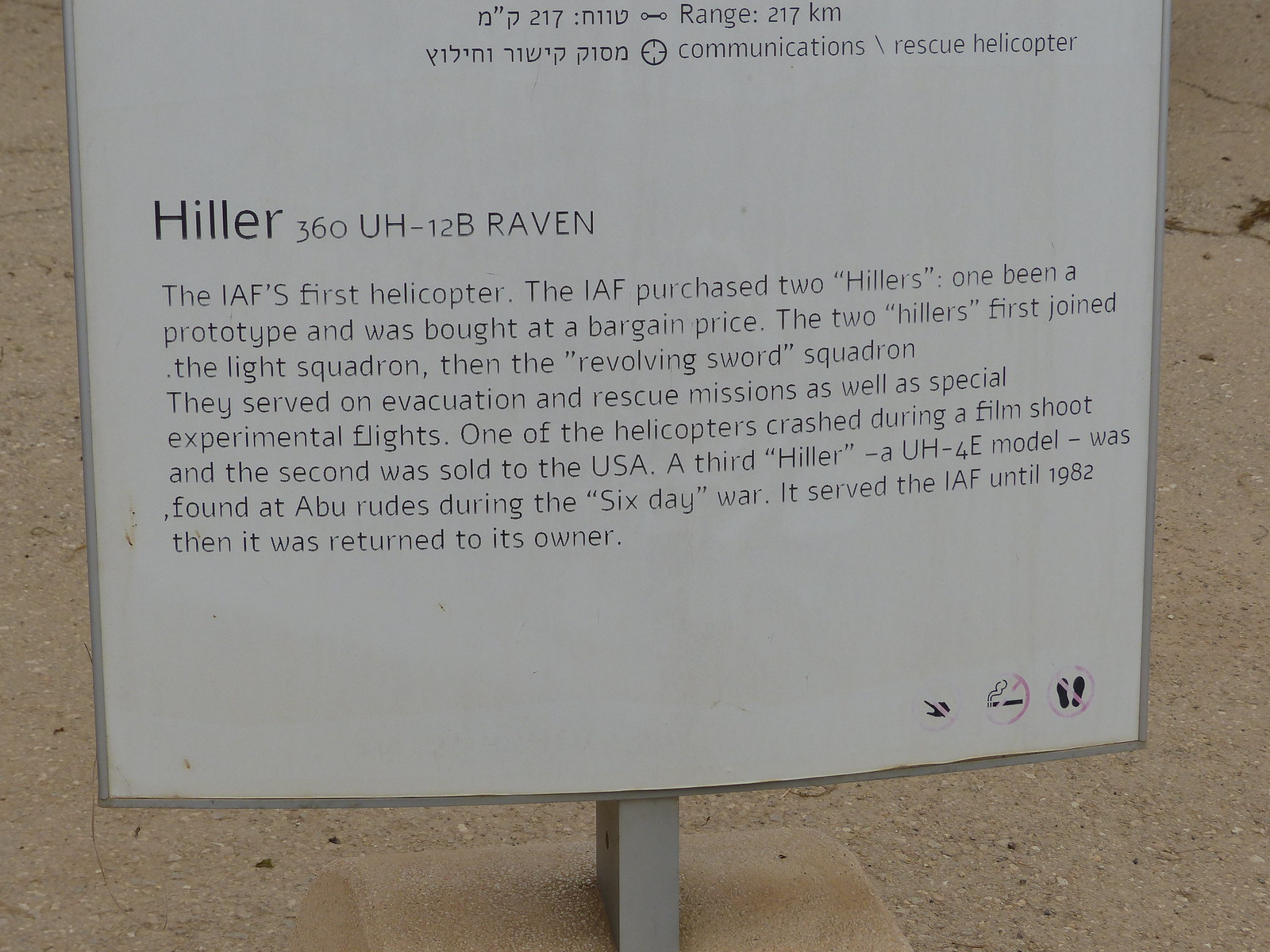The sign, likely situated at a museum or historic site, is made of metal and is mounted on a metal stand. It stands close to the ground and features white text on a black background, indicating prohibitions such as no walking, no smoking, and no touching through small icons. The text at the top is in a language other than English, followed by "Hiller 360 UH-12B Raven" written in English. The sign narrates the history of the IAF's first helicopter, detailing that the IAF purchased two Hiller helicopters, including one prototype bought at a bargain price. These helicopters were initially part of the Light Squadron and later the Revolving Sword Squadron. They were utilized in evacuation and rescue missions, as well as for special experimental flights. One crashed during a film shoot, and the other was sold to the USA. Additionally, a third Hiller, a UH-4E model, was discovered at Abu Roods during the Six-Day War and served the IAF until 1982 before being returned to its owner. The placement of the sign suggests an outdoor setting, with a dirt road or bare ground visible in the background.